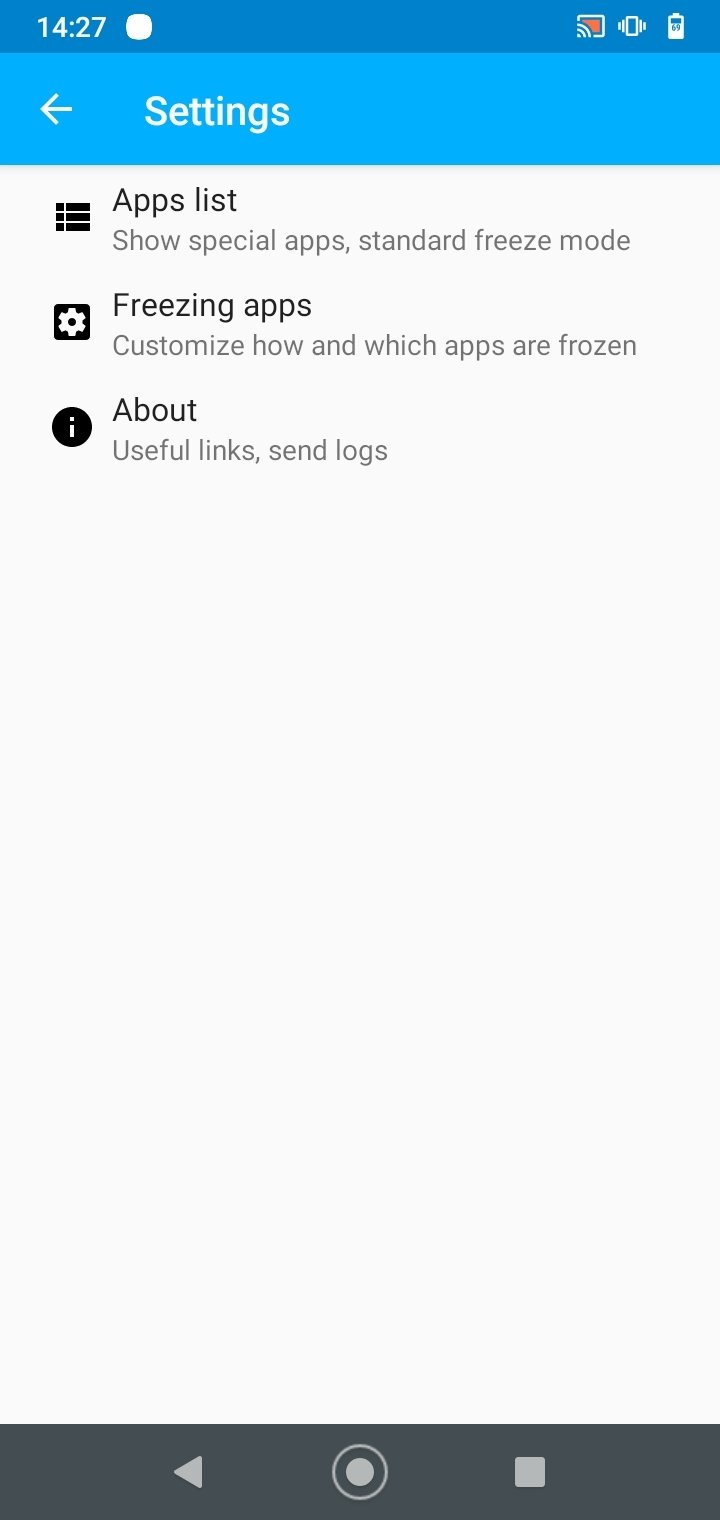A detailed mobile app screenshot of an Android device is displayed at 14:27, as indicated in the top-left corner. Adjacent to the time, there is an unusually shaped white icon, resembling a squarish circle. Following this, the interface shows the Vibrate icon, a Wi-Fi signal indicator, and a battery meter approximated to be around 28%. 

The central portion of the screenshot features a light blue background that houses the "Settings" headline, paired with a back button on its left side. Directly beneath is a predominantly white background which lists three main options:

1. **Apps List**: This section includes a dotted list format with each line item marked by a dot.
2. **Freezing Apps**: This comes with a gear icon to the left, allowing customization of app freeze settings.
3. **About**: Featuring an encircled "i" icon on its left, this section offers useful links and options to send logs.

At the bottom of the screenshot, there is a black bar containing three light gray buttons: a back button, a possible rewind button, a record button, and a stop button.